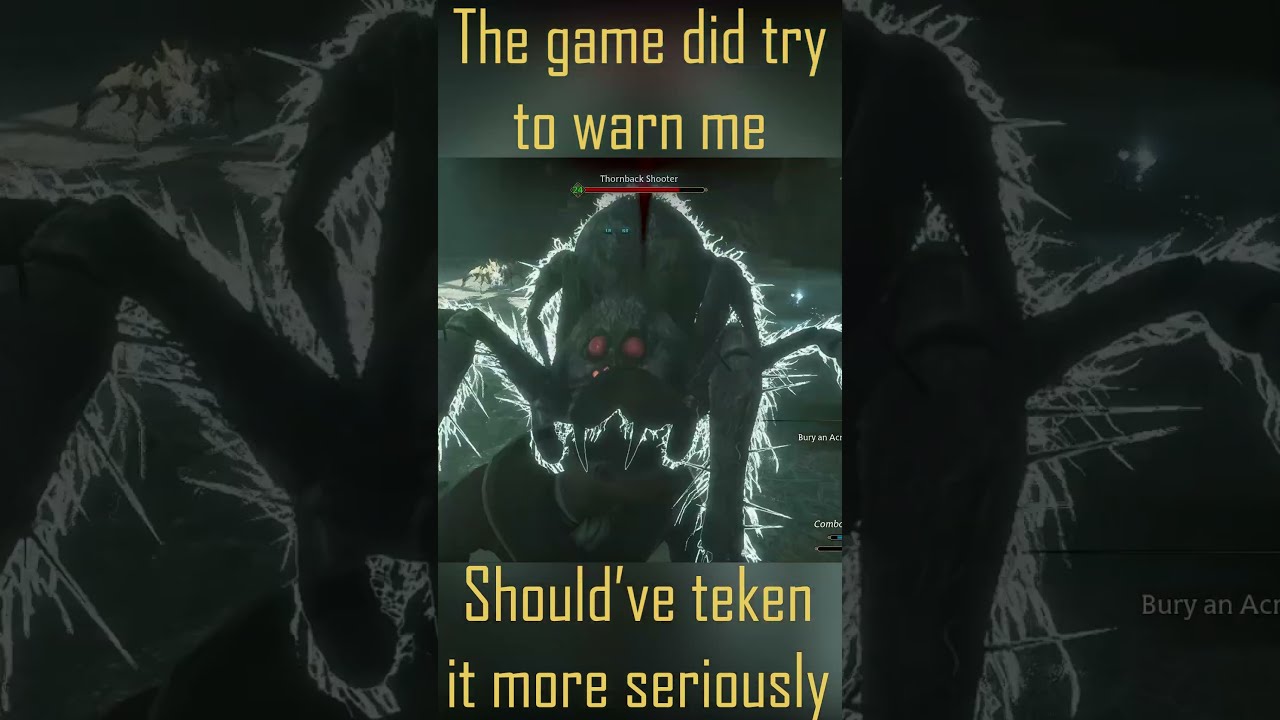In this image, we see a screenshot from a video game that prominently features a menacing, large spider attacking a character. The spider, positioned centrally, is depicted with striking detail: it has a dark, almost black body covered in white hair, and menacing, large red eyes. The spider’s hairy legs and imposing size contribute to its terrifying appearance, which is intensified by the red health bar positioned above it, indicating it’s an enemy in the game. The health bar shows minimal damage, suggesting that the battle has just begun or the spider is particularly strong. The image's background is predominantly dark, enhancing the spider's eerie presence.

Text overlays the image, formatted in a manner reminiscent of a meme, with yellow words at both the top and bottom. The top text reads, “The game did try to warn me,” while the bottom text continues, “Should have taken it more seriously.” This suggests that the player might have underestimated the threat posed by the spider. The colors in the image include shades of yellow, green, grey, white, red, and purple, which blend to create a dramatic and intense visual. All these elements combined make it a vivid and intriguing snapshot from what appears to be a mobile or social media platform game, possibly seen on TikTok or Instagram.